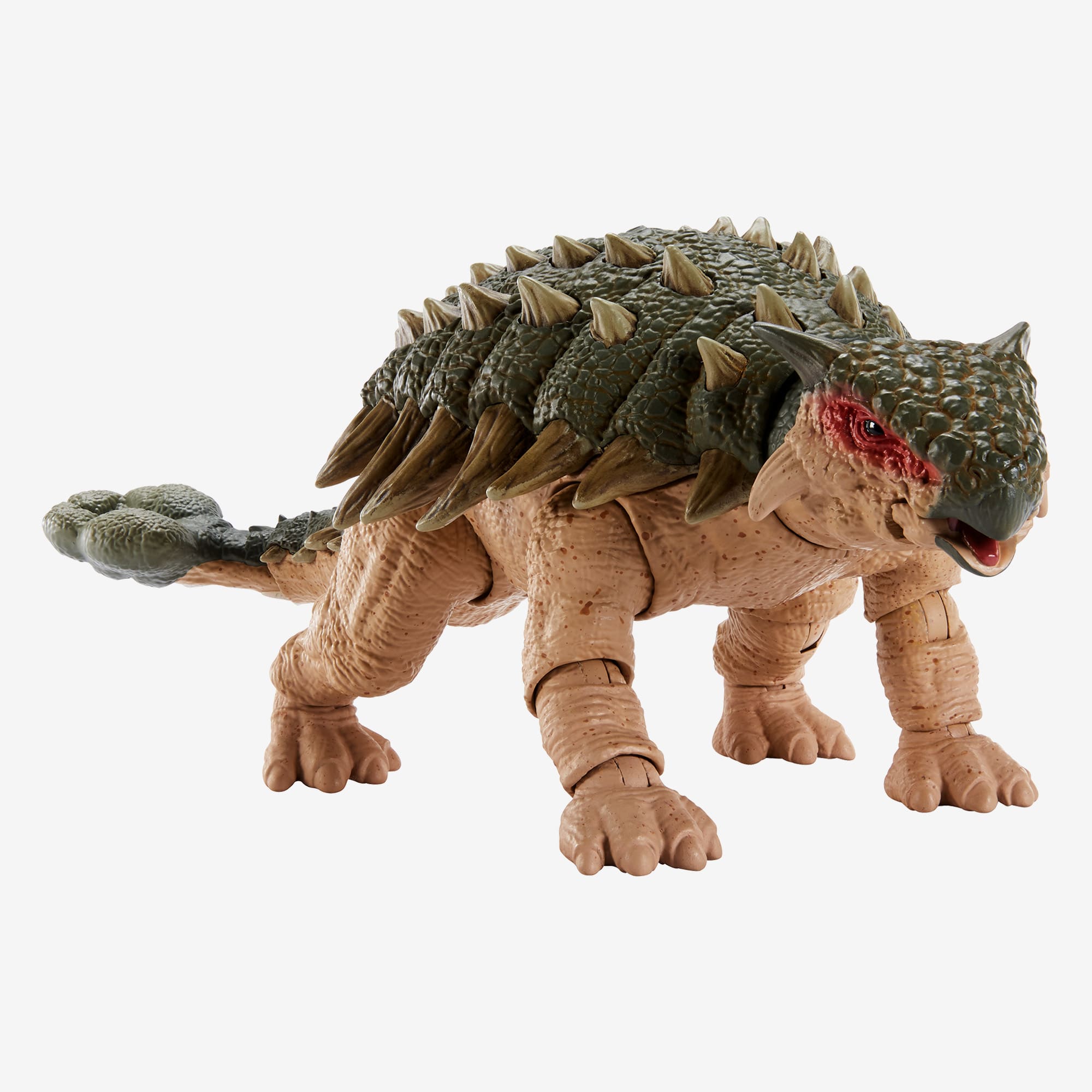The image depicts a highly detailed, plastic toy ankylosaurus dinosaur against a faint gray background. The toy, approximately six inches in both height and width, stands on all four legs with its body oriented to the right, revealing only one side of its detailed craftsmanship. The underbelly and legs, which are articulated at the knees and the upper joints, are painted a tan color speckled with brown. 

The ankylosaurus has a green head with a beaked nose and a red-streaked eye; its lone visible eye is ringed in red with a visible red tongue inside its slightly open mouth. Thorny spikes and plates cover the top part of its body, creating a rugged, bumpy texture. These spikes are grayish-brown and protrude from the areas above its eyes, cheeks, and back, mimicking armored plates. 

The toy’s head, neck, and limbs can be positioned to mimic lifelike movements, enhancing its play value. Its green, tapering tail ends in a round, clover-shaped club, mirroring the iconic defensive feature of an ankylosaurus. The model is richly detailed, with special attention given to the naturalistic texturing and coloration, reminiscent of a tortoise’s shell for the back, providing an engaging and educational representation of the prehistoric creature.